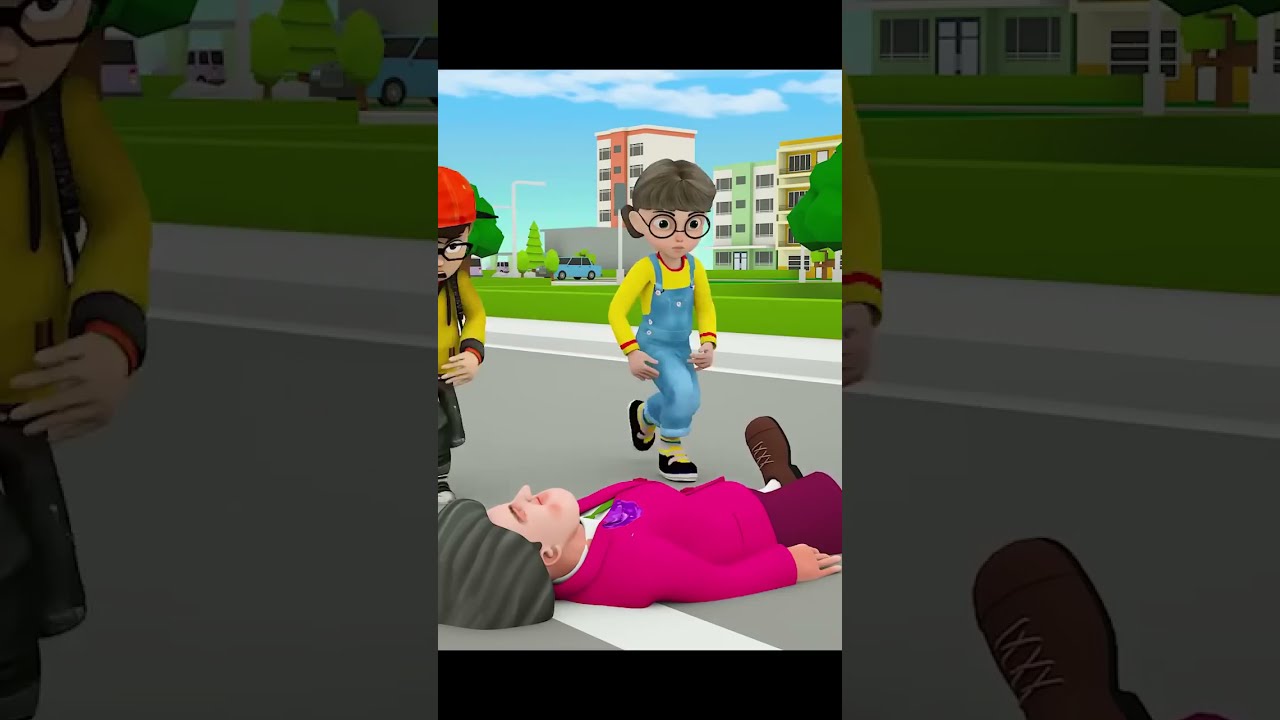This is a colorful, computer-generated image depicting a scene from a children's video game. The image is presented in a triple-frame layout, with the middle frame acting as a magnified version of the scene. At the center of this frame, an adult, possibly a woman, lies on the street wearing a magenta-colored skirt, a dark pink blazer over a white shirt, and brown shoes. Her head rests on the sidewalk, suggesting she is either unconscious or resting.

Standing over the adult is a child in blue overalls, a yellow t-shirt, and glasses with a ponytail. Next to this child, another child is partially visible, wearing black pants, a yellow top, and possibly a red or reddish-orange hat or bike helmet, with black-rimmed glasses. Both children have a shocked expression on their faces. 

In the background, one can see trees, grass, hedges, and some taller buildings, along with a couple of cars, suggesting an urban setting. The left and right frames of the image repeat parts of this scene, with the left frame showing the image larger, highlighting the shocked child in a yellow sweater prominently cut off partway, and the right frame focusing on the foot of the adult lying on the ground. The entire depiction combines a playful, cartoon style with vibrant colors to create a vivid and engaging scene.